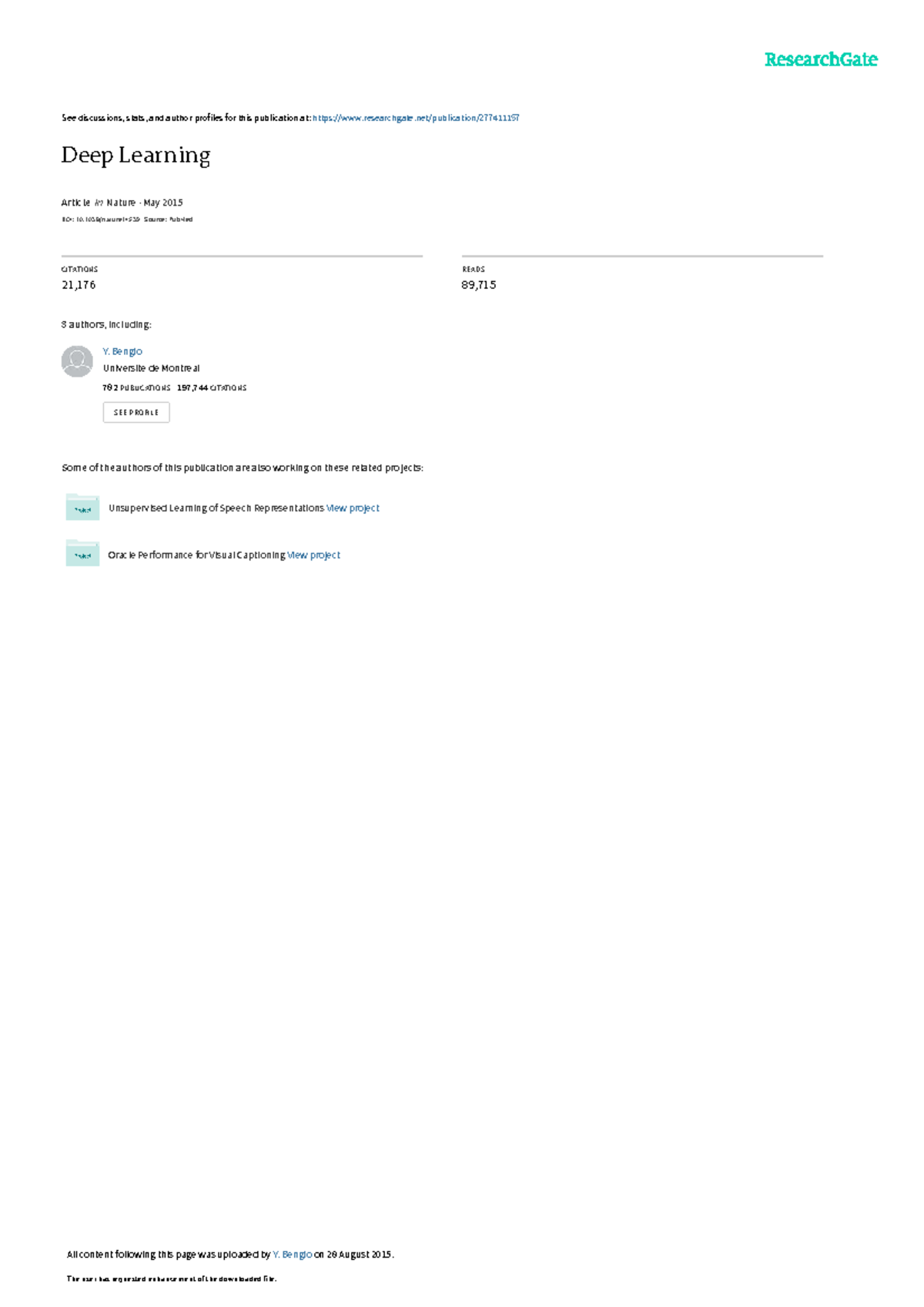This image depicts a webpage from ResearchGate. In the top right corner, "ResearchGate" is prominently displayed in green-colored text. Below it, a message reads: "See discussion stats and author profiles for this publication at" followed by a ResearchGate URL. The featured publication is titled "Deep Learning," designated as an "Article in Nature, May 2015," with its source being PubMed. The article has garnered 21,176 citations and 89,715 reads.

Three authors are noted for their contributions to this publication, including Y. Bengio from the University of Montreal, who boasts 782 publications and 197,744 citations. An option to view their profile is available.

Additionally, a section in black text indicates: "Some of the authors of this publication are also working on these related projects." Two projects are listed: "Unsupervised Learning of Speech Representation" and "Oracle Performance for Visual Captioning," each with a blue text link to view the project.

At the bottom of the page, a note states: "All content following this page is uploaded by Y. Bengio on the 28th of August, 2015," followed by: "The user has requested enhancement of the downloaded file."